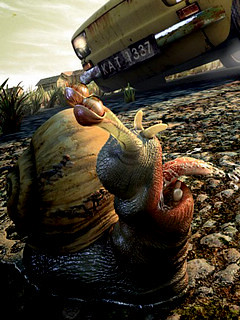In the image, we see a detailed computer-generated scene depicting a whimsical garden decoration. Dominating the foreground is a vividly animated snail figurine. The snail, with a yellow-brown shell, has a green body that features a red mouth with a bumpy pink tongue sticking out. This quirky character has large, expressive googly eyes atop long antennae, which end in round tips. The snail is positioned on a gravelly surface amidst larger rocks. 

A notable element in the background is an old yellow car with its headlights on, sporting a European-style black license plate reading KAT1337. The car appears slightly uphill and in disrepair. Surrounding the scene, we can glimpse a few blades of grass, various plants, and further in the distance, a gray-roofed house. The overall setting evokes a charming and slightly surreal atmosphere.